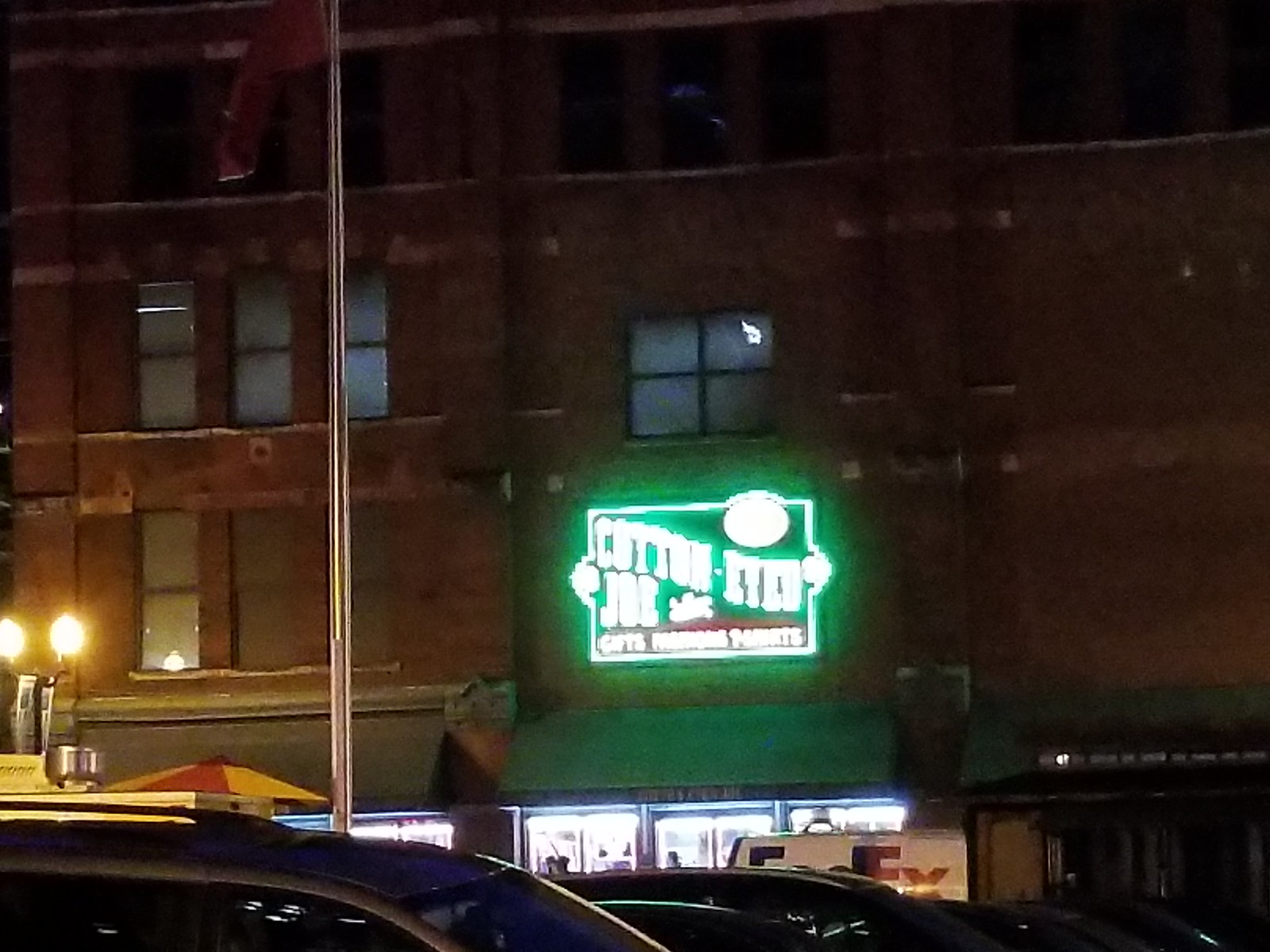As you approach the eatery, you snap a photo from the sidewalk, capturing the establishment's green sign, partially obscured but suggestive of a restaurant or bar. On the left, several flagpoles stand prominently, hinting at a sense of pride or decoration. The foreground is dominated by the sleek hoods of around four to five parked cars, indicating bustling activity. A FedEx truck is also parked conspicuously in front of the building, emphasizing the urban environment. The structure of the venue itself appears to be connected to an adjacent building, framing the scene within a typical cityscape.